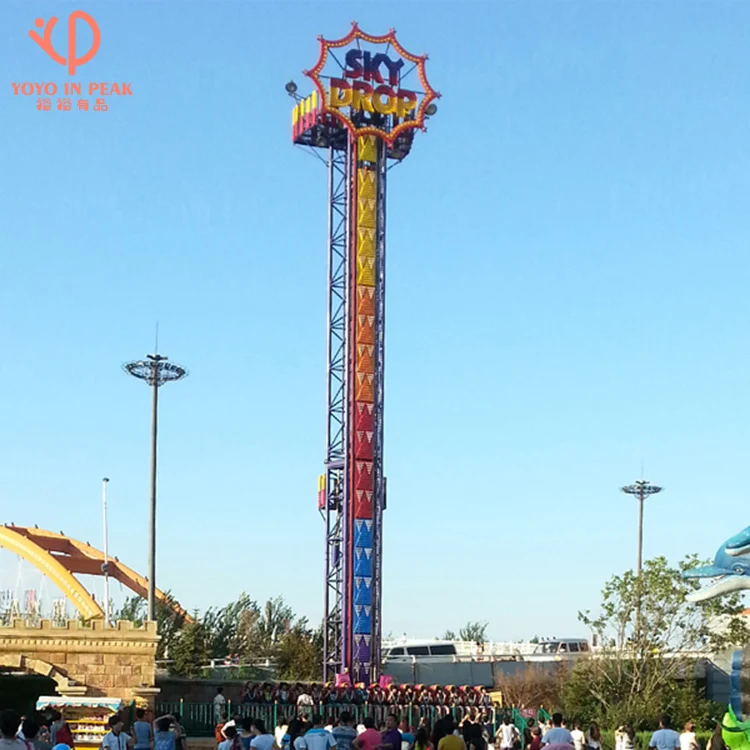In this vibrant daylight photograph of an amusement park, the centerpiece is the towering Sky Drop ride featuring an eye-catching design with a burst-like appearance at the top in bright blue, red, and yellow. This striking ride transitions in color down the stalk from yellow to orange, red, and finally blue at the base. It stands tall amidst a backdrop that includes other carnival rides, some speakers on poles or spears pointing skyward, and a clear, cloudless sky. To the left, there's a bridge-like structure, while the bottom left corner reveals a structure resembling a castle. On the bottom right, there is a dolphin figure with its mouth open. The foreground is filled with numerous park-goers walking to and from the ride, their backs turned to the camera. The upper left-hand corner features text that reads "Yo-Yo and Peak," accompanied by some unidentifiable symbols.